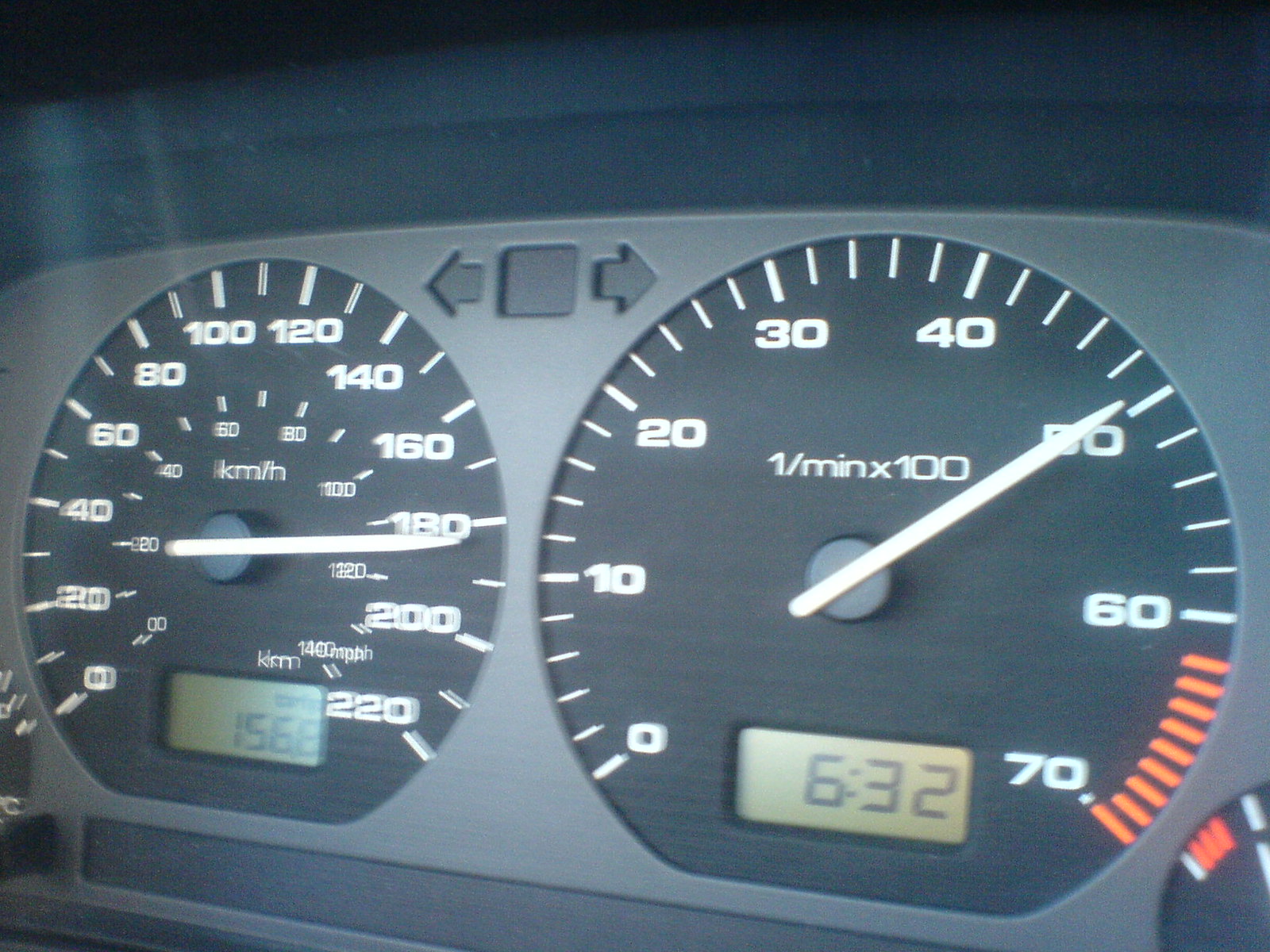The image depicts the front dashboard of a car, focusing on the instrument cluster situated behind the steering wheel. The centerpiece of the cluster displays two prominent black circular gauges against a grayscale and black background. 

The first gauge, located on the left, is a speedometer that features both kilometers per hour (km/h) and miles per hour (mph). The gradations on this dial range from 0 to 220, with the major markings at 100 and 120 positioned towards the top. The numbers are displayed in a clear, white font. A white needle indicates the current speed, pointing just above the 180 km/h mark. At the very top of the speedometer gauge, between the two black sections, lies a small square flanked by two arrows.

The second gauge, found on the right, is a tachometer calibrated from 0 to 70, with the numeral increments representing 1 x 100 revolutions per minute (RPM). Notably, the section beyond 60 is highlighted with a series of red markings, extending all the way to 70, while the remaining markings are in white. The needle on this gauge is currently pointing towards the 50 mark. Additionally, there's a digital readout showing the time "6:32," likely indicating the current time of day.

The image is slightly blurry on the left side, and there are noticeable shadows and light reflections adding depth to the scene, emphasizing the three-dimensional aspect of the dashboard.